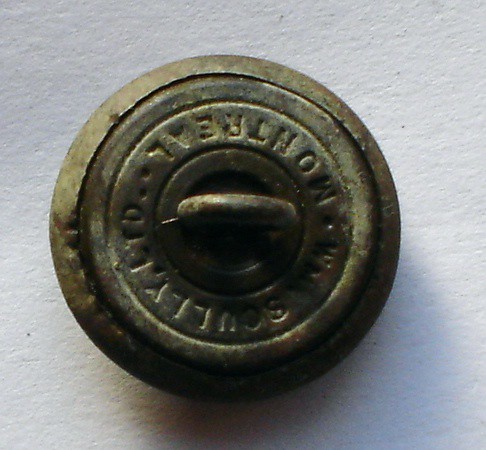The image depicts a weathered and rusted round object that resembles a button, but without the holes. It features a slightly raised ridge around the edge that appears somewhat detached, hinting at its age and wear. The object is primarily rusted and displays shades of brown, green, gray, and black.

At the center of the object, there is a horizontal mark, possibly indicating a handle or pull, as it bears a slight resemblance to a drain cap. Surrounding this central area, indented or engraved lettering is visible, although upside down in the image. The text reads "Scully Ltd." around the bottom right curve and "Montreal" spanning from the top right. It also includes two letters that are unclear.

The round item is placed on a white surface that might be plaster or some other material, suggesting it is resting on a table or similar flat surface.